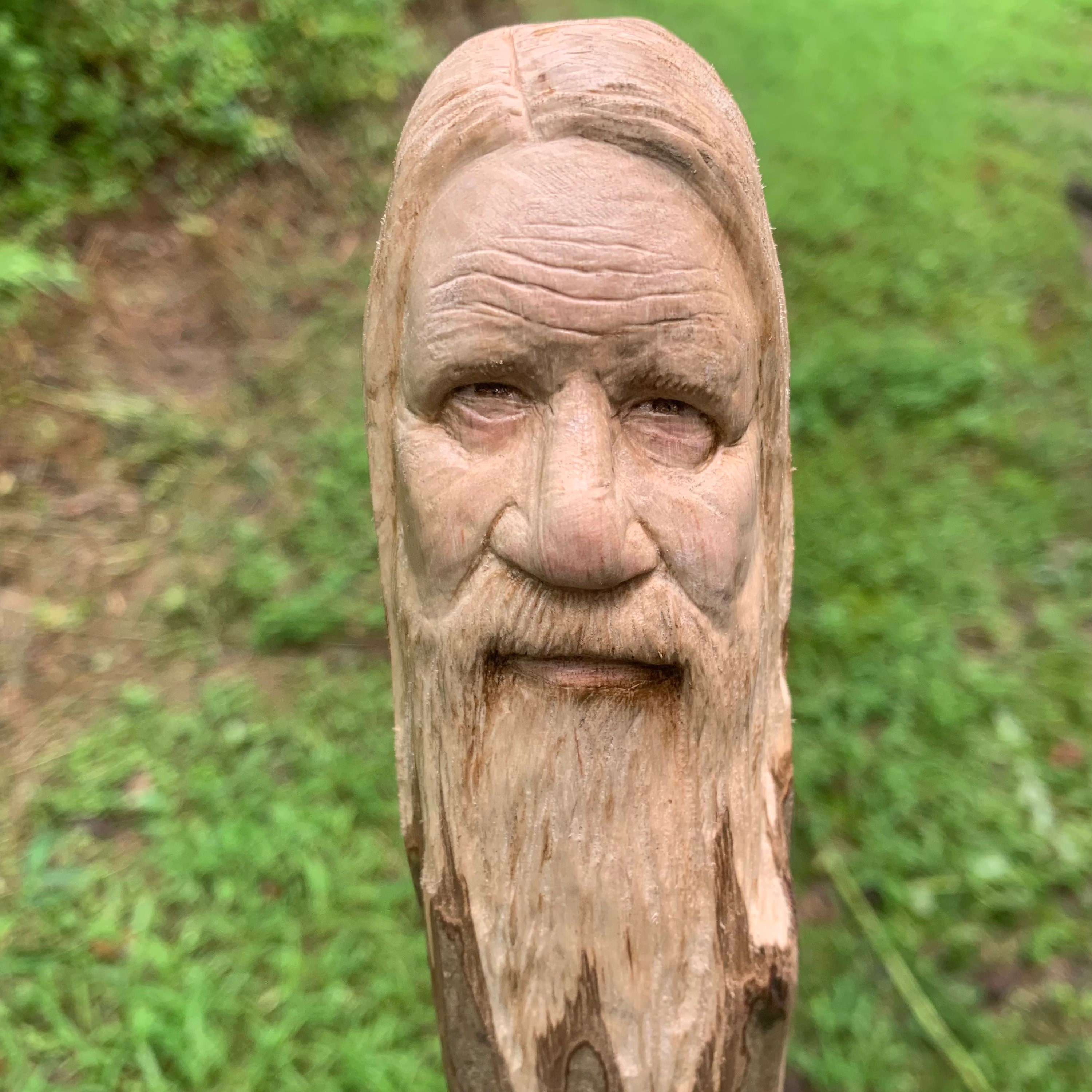The photograph showcases an intricately carved wooden sculpture set against an outdoor backdrop. The background features a combination of grass, dirt, and what appears to be a bush in the upper left corner, though it might be overgrown grass. The wooden carving itself depicts an elderly man with a notably unfinished lower portion, where the beard seamlessly merges into the uncarved wooden bark. The sculpture is mounted on a pole, roughly the width of a human arm.

The man's face is exquisitely detailed, complete with kind eyes, a larger nose, a mustache, and a full beard. His hair is parted to the right and falls long down the sides of his head. The man exudes a serene and relaxed demeanor, highlighted by his gentle smile and the worn lines on his forehead, indicative of his age. The craftsmanship is exceptional, capturing the essence of an older man with striking realism. The carving evokes a sense of wisdom and tranquility, reminiscent of mythological figures, though the man has both eyes, differentiating him from deities like Odin. This finely detailed piece stands out as a remarkable example of traditional wooden artistry, not commonly seen.